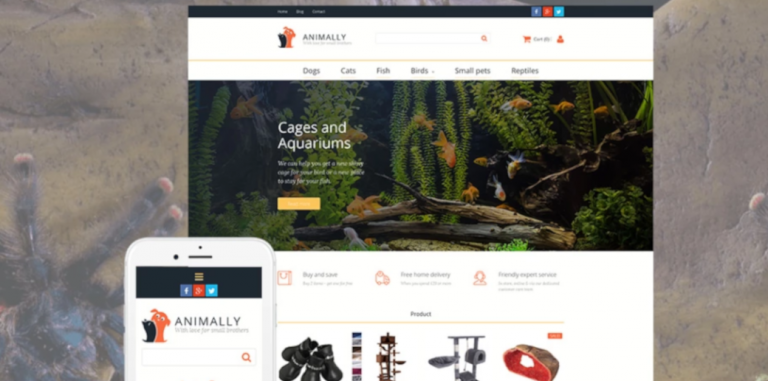Catalog Page from Animally - Featuring a Vibrant Aquarium

The image showcases a section of a catalog from a company called Animally. The logo, positioned prominently, features a cartoonish brown puppy with its head tilted to one side and a black cat sitting in front of it, appearing to look at its feet. This logo is against a backdrop of a circular design, enhancing its visual appeal.

In the center of the webpage, there is a captivating picture of a well-maintained aquarium teeming with life. The aquarium is home to various goldfish and other multicolored fish, all gracefully swimming amidst lush green weeds, ornamental branches, and natural rocks placed at the bottom. The vibrant colors and dynamic composition create an enchanting underwater scene.

Accompanying the image is a small yellow rectangle, possibly a clickable button designed to interact with the aquarium picture, perhaps to enlarge it or provide additional details.

Below the aquarium image, the Animally logo is reiterated, this time in a slightly larger format for emphasis. The page is organized with headings for different categories of pets: Dogs, Cats, Fish, Birds, Small Pets, and Reptiles, making it easy for users to navigate through the catalog.

At the bottom of the screen, various pieces of pet-related equipment are depicted, likely to provide users with options for enhancing their pets' habitats and ensuring optimal care. Overall, the page is visually engaging and thoughtfully organized, catering to pet enthusiasts and their diverse needs.